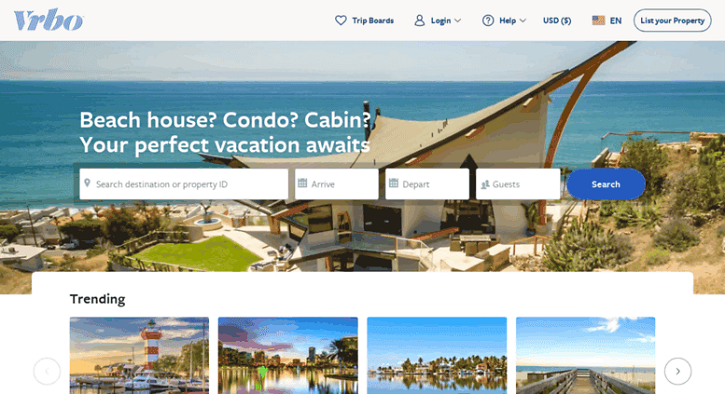This image showcases a section of the Vrbo website interface. At the top of the screen, the heading features 'Vrbo' in blue lettering, complemented by a grey font. On the right side, a blue heart icon labeled 'Trip Boards' is visible. Adjacent to it, another image displays a circular icon representing a user's head and shoulders, with an adjacent dropdown arrow for the login menu. Further to the right, there is a blue question mark in a blue circle labeled 'Help', followed by a grey dropdown arrow next to 'USD', and an American flag icon indicating the currency option. 

The 'EN' option in blue denotes the language settings. To the right, a blue circle with blue lettering invites users to 'List Your Property'. Below, a scenic photo depicts a beach destination with a grey sky and blue water. On the left side of this image, white font highlights potential vacation types: "Beach House? Condo? Cabin? Your perfect vacation awaits."

A white search box below this prompt includes fields such as "Search destination or property ID" in grey font. Additional fields include 'Arrive' and 'Depart', each accompanied by a calendar icon, and another field for 'Guests' with head and shoulder icons. A blue 'Search' button is located beside these fields.

Below this section is a white box with the heading 'Trending' in black font. A grey circle at the bottom contains four images, showcasing different scenic views: a boat pier, a waterfront with buildings against a blue sky, a neighborhood with houses and trees under a blue sky, and a beach with a grey wooden boardwalk. Adjacent to these images is a grey circular arrow pointing to the right.

Lastly, located above this section is an image of a house featuring a grey roof, brown wooden beams, and green elements on the left. There is a beach property behind it, with trees and bushes on the right, as well as a railing and what appears to be the white base of the house.